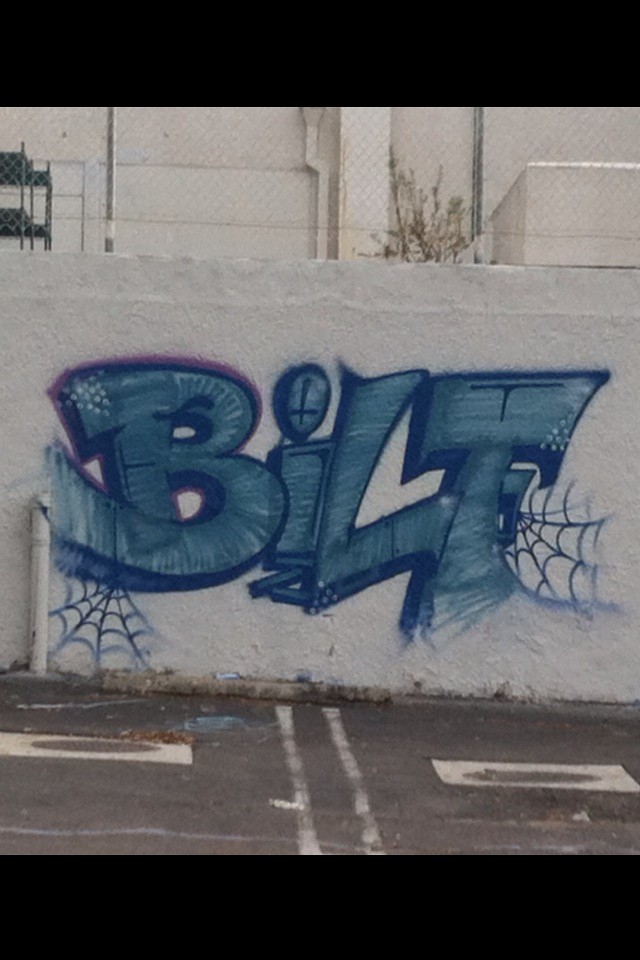The image captures a pristine white wall, likely made of brick or stone, situated alongside a parking lot. The wall is adorned with distinctive blue graffiti that spells out "B-I-L-T" in a very artistic and fancy font. The letter 'I' is lowercase while the other letters are uppercase, all in block lettering. The blue spray paint gradually transitions from light to dark towards the edges, adding depth to the artwork. Intricate designs, including spiderwebs, extend from the bottom of the 'B' and the side of the 'T', giving the text an elaborate, somewhat whimsical appearance. The wall is bordered by white lines marking two parking spaces on the ground below, and a tree along with a small gate is visible above the wall, enhancing the urban setting.